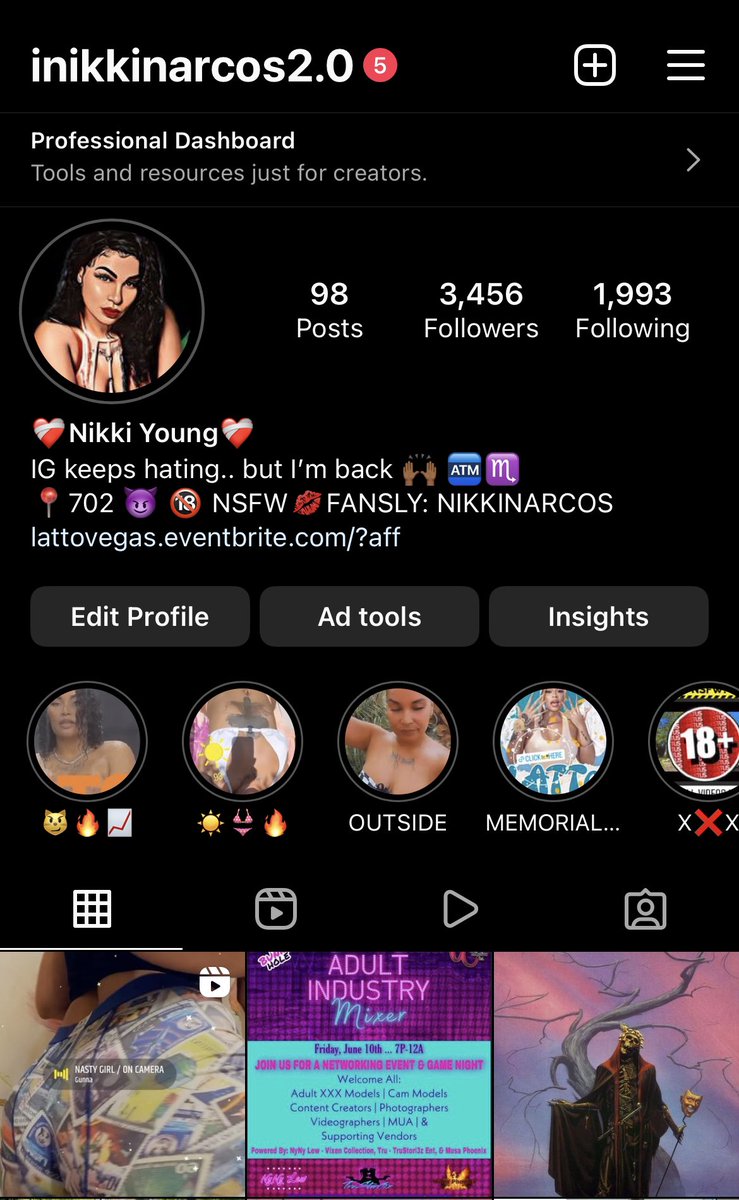Here’s a detailed and cleaned-up caption for the described image:

---

The image depicts a social media profile with a dark-themed interface. At the top left corner, in white letters against a black rectangle, it reads "INIKKINARCOS2.0" and beneath it, "Professional Dashboard." Below this section, there is a circular animated photo of a woman with black hair. Her name, "Nikki Young," is written with a red star on either side. Adjacent to her photo, the statistics are displayed in white letters: "98 posts," "3,456 followers," and "1,993 following." 

Underneath her name, a personal message reads: "IG keeps hating but I'm back." Further down, within a black triangular section, three options are listed from left to right: "Edit Profile," "Add Tools," and "Insights."

The next section features five circles, each containing different photos:
1. A woman in an orange outfit with black hair.
2. A picture of a tattoo.
3. A woman with brown skin wearing a black and white outfit.
4. A man wearing a white tank top.
5. An icon labeled "18+" with "XXX" beneath it, where the middle "X" is red and the other two are white.

Below these circles are three smaller photos:
1. An indistinct part of a person's body.
2. A picture with text reading "Adult Industry," deemed inappropriate.
3. An image resembling a video game character holding an object, with a background featuring lightning bolt-shaped elements that look like a tree trunk.

---

This caption provides a vivid and organized description of the social media profile as described.